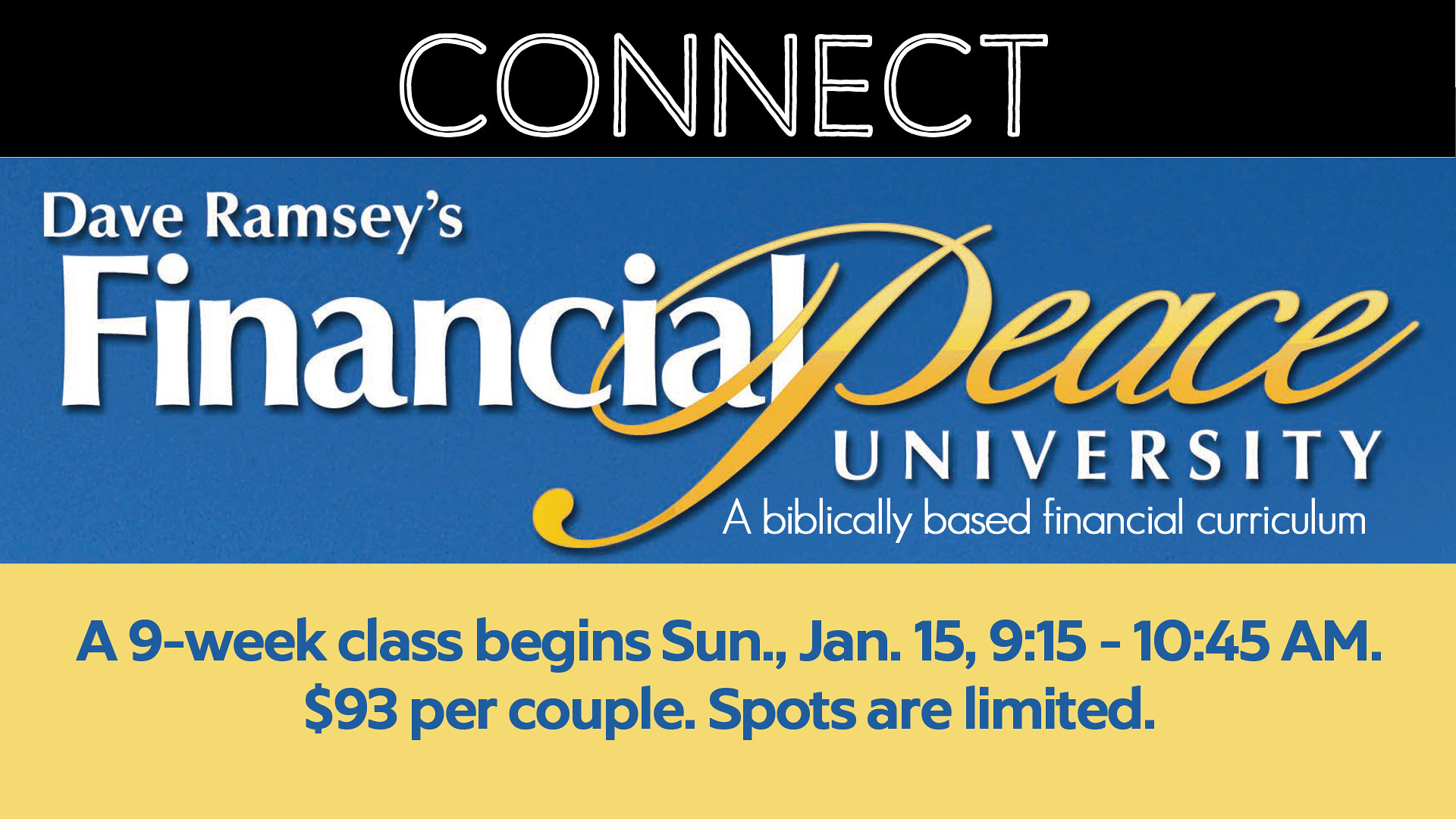The image is an advertisement for Dave Ramsey's Financial Peace University. At the top, a black rectangle with white text reads "CONNECT." The center portion of the image, shaded in a grayish-blue, prominently displays the program's title: "Financial Peace University." Here, "Financial" and "University" are in white text, while "Peace" is written in gold cursive, with the capital P's swirl artistically wrapping around the letters I, A, and L. This section emphasizes the biblically based financial curriculum offered. At the bottom, a strip of bright yellow contains dark navy blue text providing details: "A nine-week class begins Sunday, January 15th, 9:15 - 10:45 a.m. $93 per couple. Spots are limited."